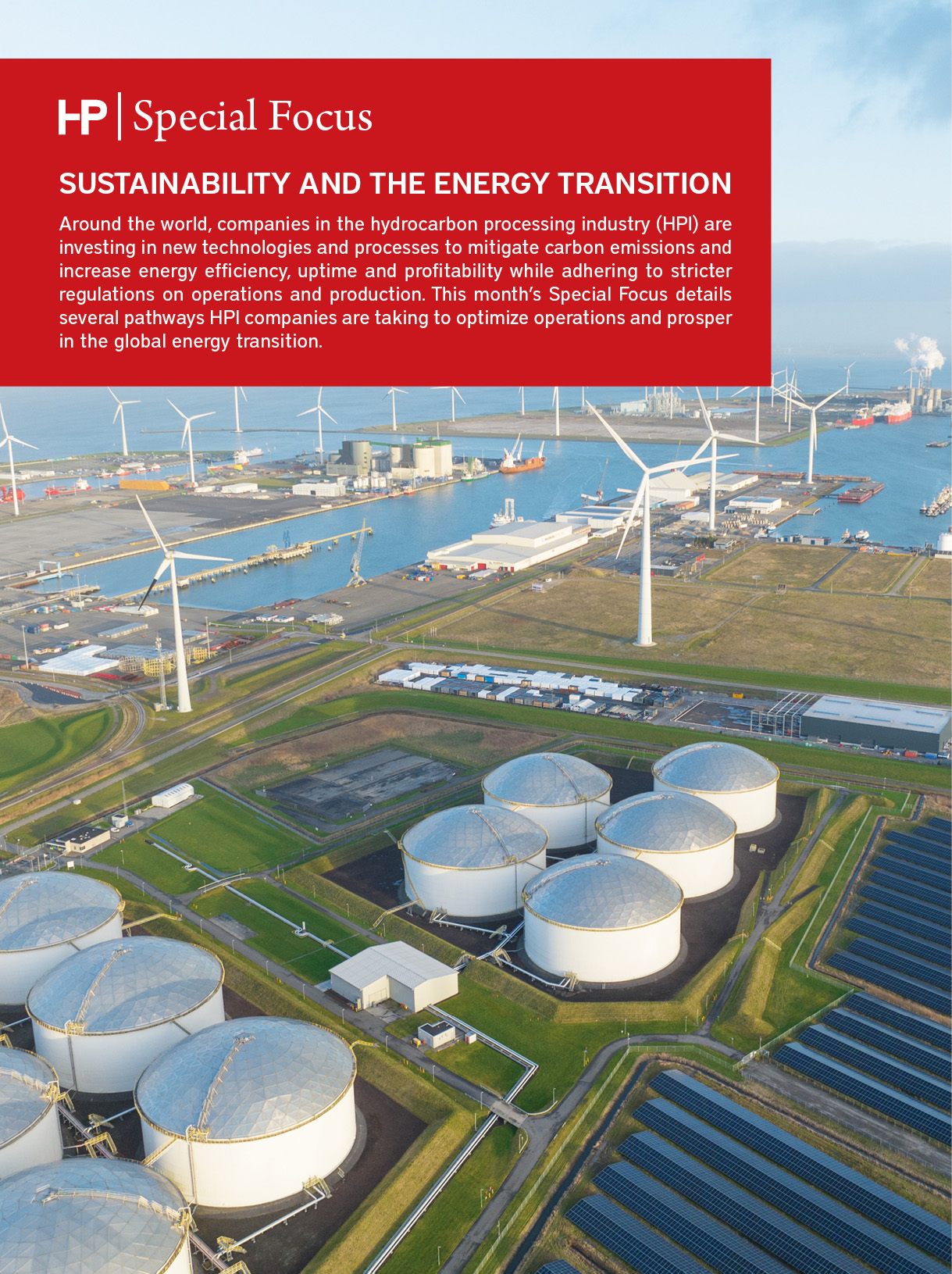An overhead aerial photograph captures a striking contrast between a tank farm and a wind power farm. In the upper left-hand corner, a red box with white text reads "HP Special Focus: Sustainability and Energy Transition," accompanied by a descriptive paragraph detailing the scene below. Dominating the bottom left and center of the image are several large, white cylindrical tanks with domed tops, set amidst expanses of green grass. Further in the distance, a vast body of water extends, potentially an ocean, with piers stretching out into the blue expanse. These piers are crowned with towering white windmills that have sleek posts and propeller blades. Surrounding these wind turbines are large, white buildings and parking lots filled with cars. Above, a serene blue sky dotted with clouds enhances the juxtaposition of the industrial and renewable elements within this landscape.